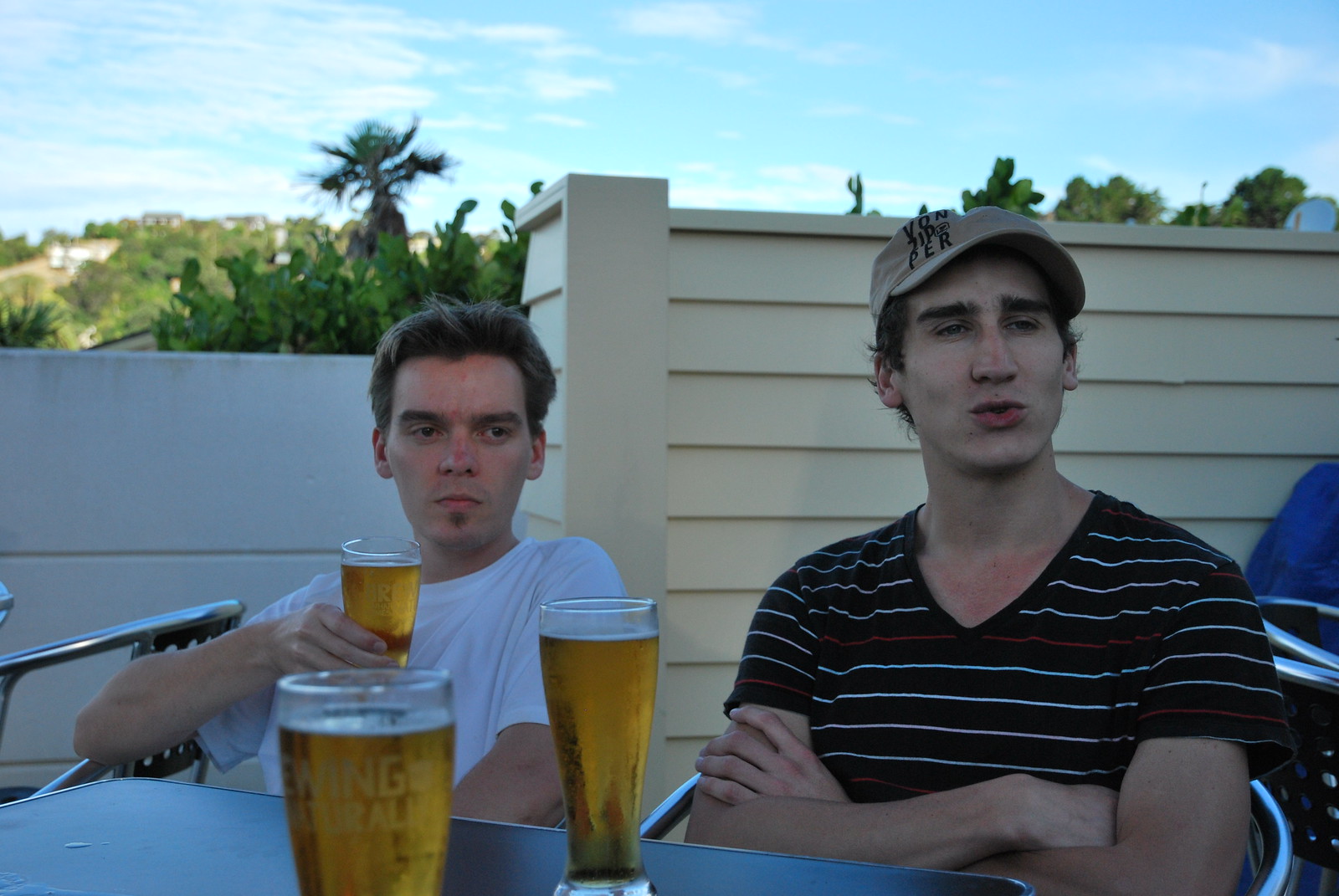In this detailed outdoor image, two young Caucasian men are seated at a table, basking in what appears to be a clear, bright, and sunny day. On the table, there are three full glasses of draft beer. The man on the left, sporting brown hair and wearing a plain white t-shirt, holds a beer glass in his right hand. His mouth is closed as he looks slightly to his right. Seated beside him, the man on the right is dressed in a black t-shirt with red and white stripes and a brown baseball cap, his arms crossed and his lips pursed, seemingly caught mid-sentence. Both men gaze to their left, suggesting they're engaged with an off-camera person, who might own the third beer on the table. Behind them, a white wall merges into a taller beige wall, framed by the lush green leaves of plants. In the far distance, a hill and a palm tree stand against a backdrop of a blue and white sky. The scene conveys a relaxed atmosphere, likely at an outdoor bar or café.